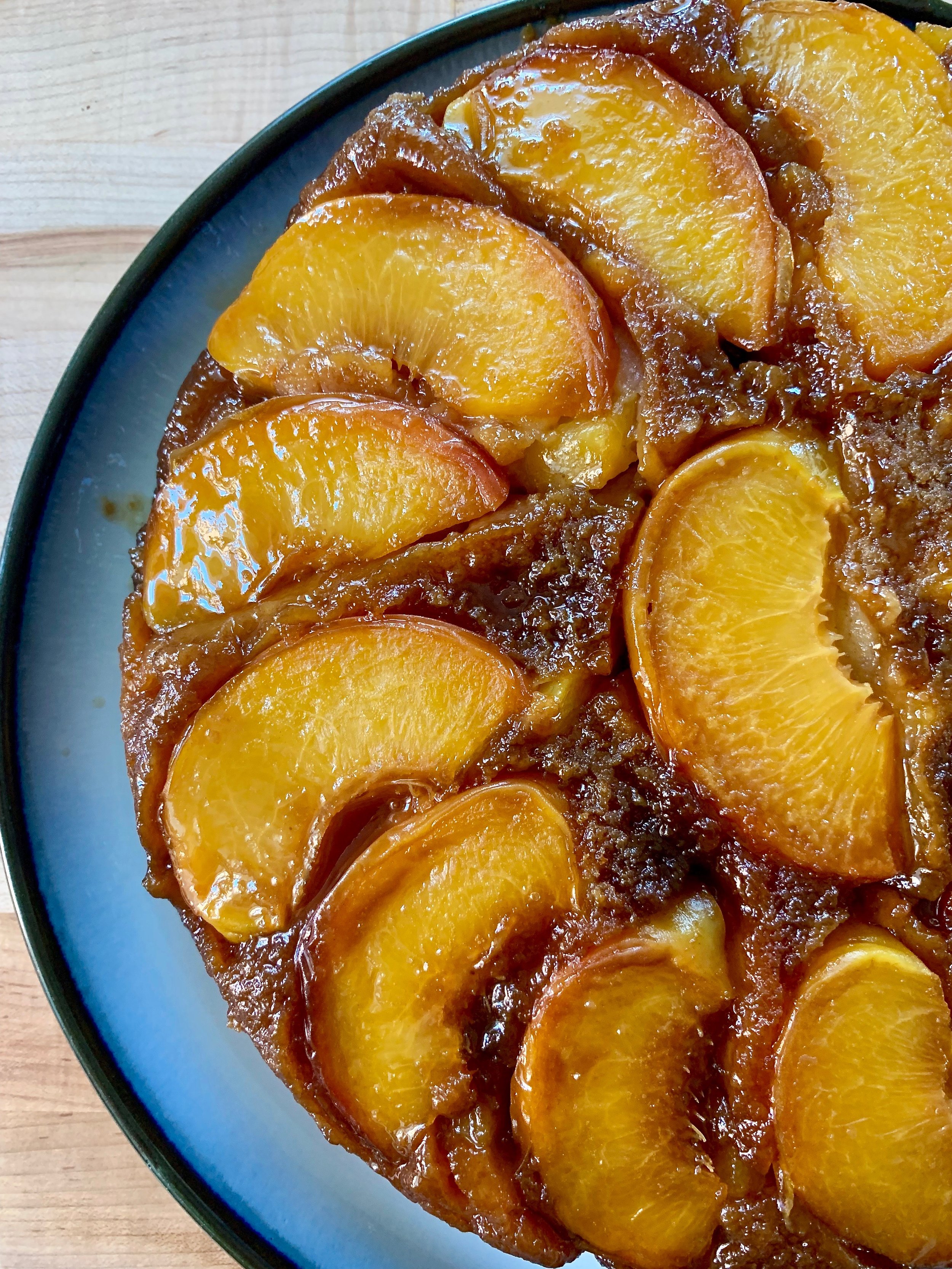This is a detailed color photograph of a baked peach dessert reminiscent of a pineapple upside-down cake, presented on a table. The dessert is displayed on a circular blue plate with a dark blue border and a medium blue interior, which is half-visible in the image, forming a semi-circle. The background features a light faux wood surface with horizontal striations akin to tree bark. The dessert comprises sliced peaches arranged in a pattern, nestled closely together in a thick, sugary brown sauce. The peaches are flat, with edges that are dark brown from baking. The syrupy texture suggests they were likely fresh before baking and the dessert has an appealing gooey appearance. The arrangement and presentation indicate it might have been prepared for a visual display, like an online recipe blog or a cookbook.